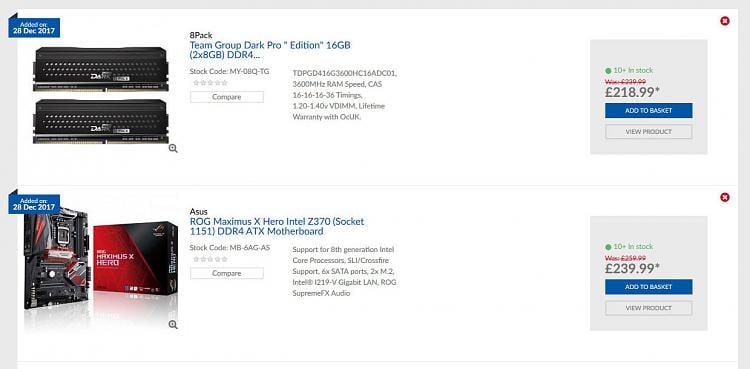This image features two items displayed in their original packaging. The first item is an 8-pack of Team Group DAC Pro Trademark Edition DDR4 RAM, offering a total of 16GB through two 8GB modules. This product, identified by the stock code MyOBQTG, was included in the inventory on December 28th, 2017. The second item is an ASUS ROG Maximus X Hero motherboard, designed for Intel's 8th Generation Core processors. This ATX motherboard utilizes the Z370 chipset and supports features such as SLI and Crossfire for multi-GPU setups. It offers six SATA ports, two M.2 slots, Intel's 1219V Gigabit LAN, and ROG SupremeFX audio for superior networking and sound quality.